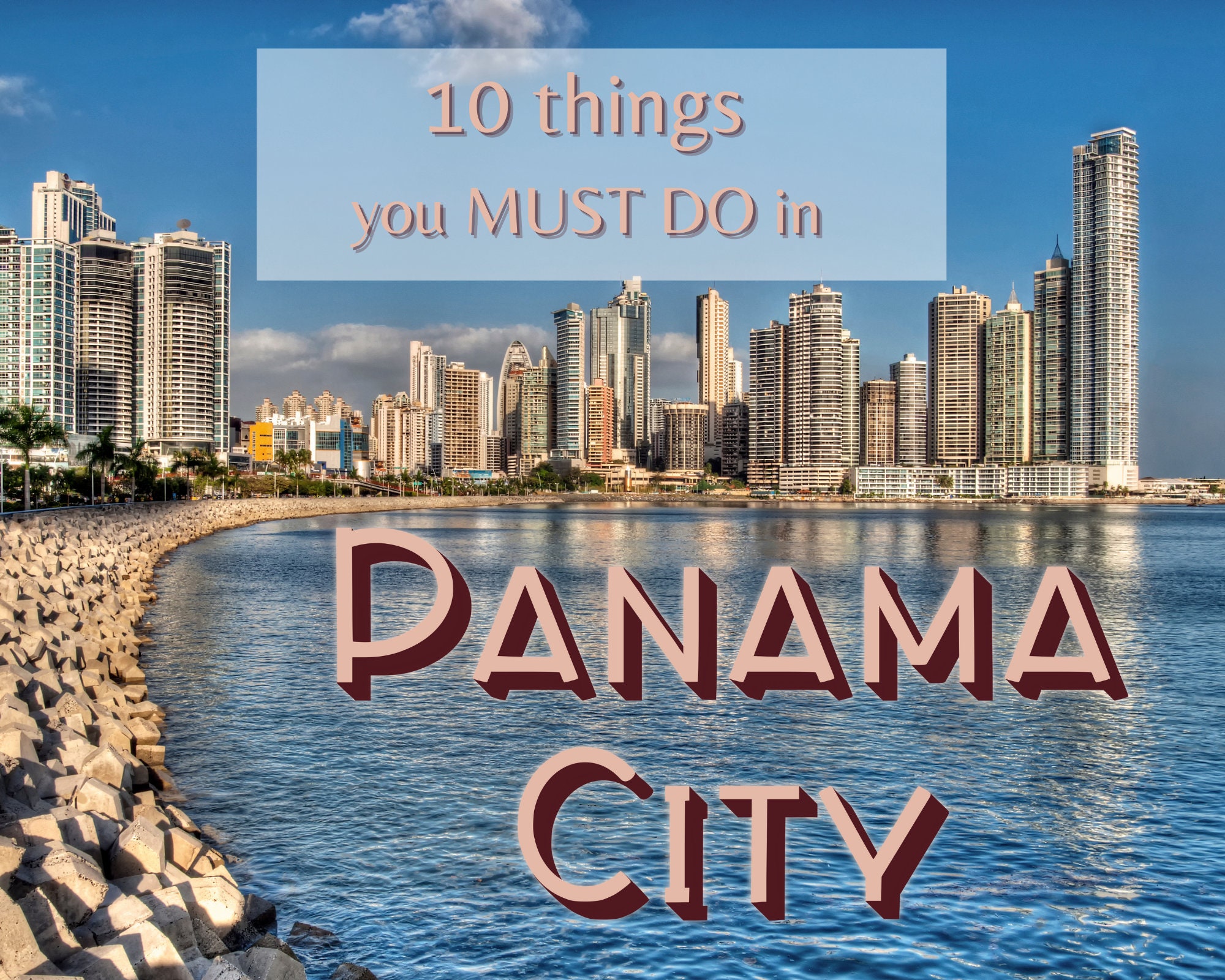The image features a vibrant, daytime photograph of Panama City with a striking overlay of text at the top and bottom. At the top, inside a light blue rectangle, the eye-catching pink text reads, "10 things you MUST do in," formatted with "MUST" capitalized for emphasis. Dominating the bottom of the image in large, bold capital letters, the phrase "PANAMA CITY" stands out prominently.

The backdrop showcases Panama City's impressive skyline, with numerous whitish-gray buildings ranging from medium height to towering structures, some extending dozens of stories high. These buildings likely serve as office spaces or apartment complexes. In the foreground, there's a serene body of water bordered by a rocky shoreline, devoid of any beaches. Scattered palm trees can be seen beyond the rocky shore, adding a tropical touch to the urban scene.

The sky above is a clear, even blue accented by a scattering of clouds, indicative of the pleasant daytime weather conditions in which the photo was taken. The shoreline appears tranquil, with no visible people or boats, and only a few indistinct vehicles in the distant background. This peaceful, urban waterfront scene captures the essence of Panama City’s dynamic yet relaxed atmosphere.